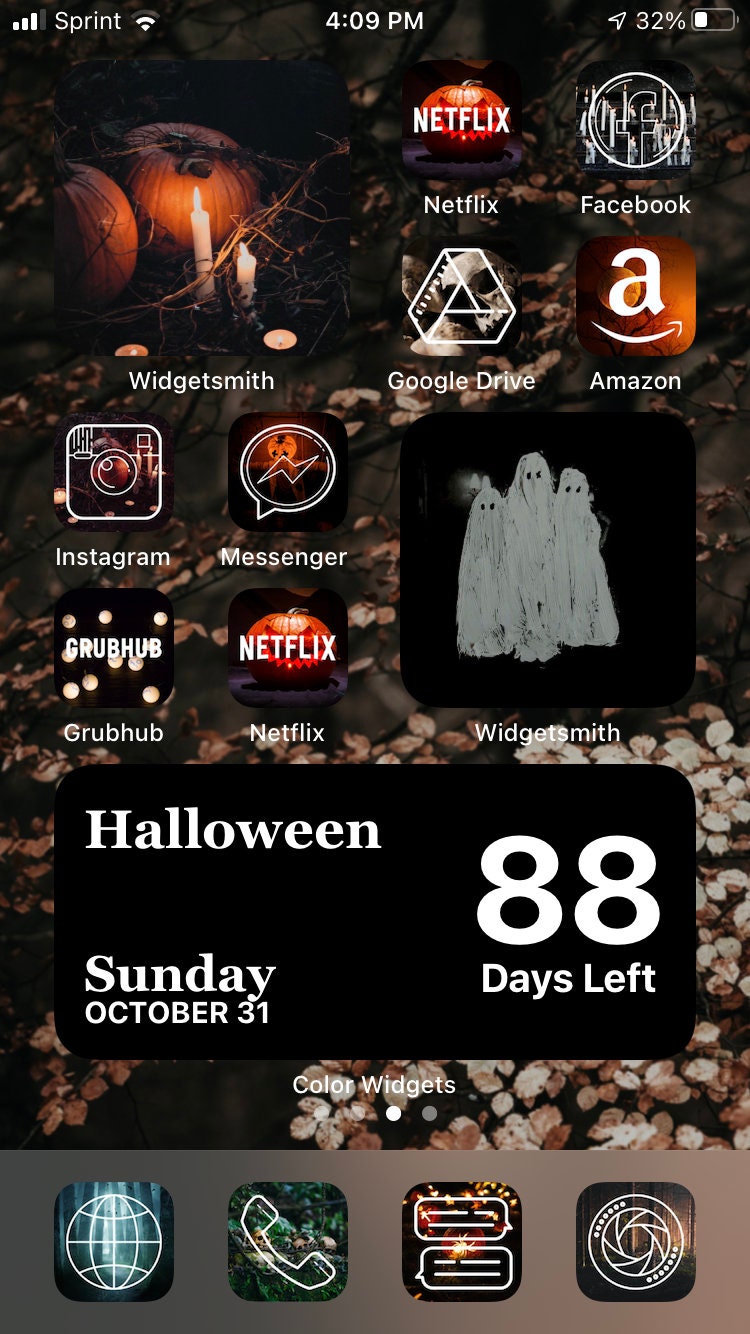The image depicts a smartphone screen with a Halloween-themed wallpaper. The background showcases a dark, eerie scene adorned with jack-o'-lanterns, circular leaves, and coins, contributing to the spooky atmosphere. Prominently displayed on the screen is a small rectangular widget that announces "Halloween Sunday, October 31," followed by a countdown of "88 days left," emphasizing the Halloween theme. The application icons on the screen are also customized to fit the Halloween motif. The Netflix icon features a pumpkin face instead of the traditional logo, and the Facebook icon appears hand-drawn, resembling a pencil sketch. Other visible app icons include Google Drive, Amazon, Instagram, Messenger, Grubhub, Netflix, and Widgetsmith. At the bottom of the screen, the traditional icons for internet browsing, phone calls, messaging, and settings are also present.